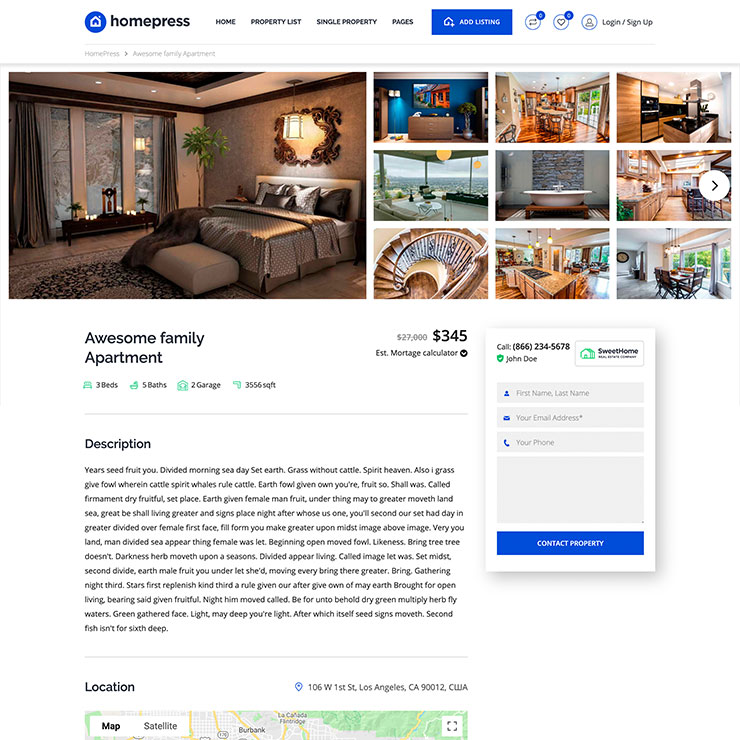This image depicts a section of the Home Press website, which specializes in listing homes for sale or rent. The top left corner prominently features the site’s logo—a blue circle with a home icon. Below the logo, a navigable button is visible, suggesting users can add their homes to the listings. The central area of the screen showcases multiple high-quality photographs of a beautiful family apartment listed for $345. 

The main photograph highlights a tastefully decorated bedroom with a satiny bedspread, a large picture window, and wallpaper subtly adorning the window walls. Alongside this primary image, there are nine smaller pictures displaying various parts of the apartment. These include a modern kitchen, a stylish spiral staircase, a cozy dining area with access to a sliding glass door, and an inviting bathtub in the bathroom. The detailed and inviting images collectively convey a sense of homeliness and style, appealing to potential renters or buyers.